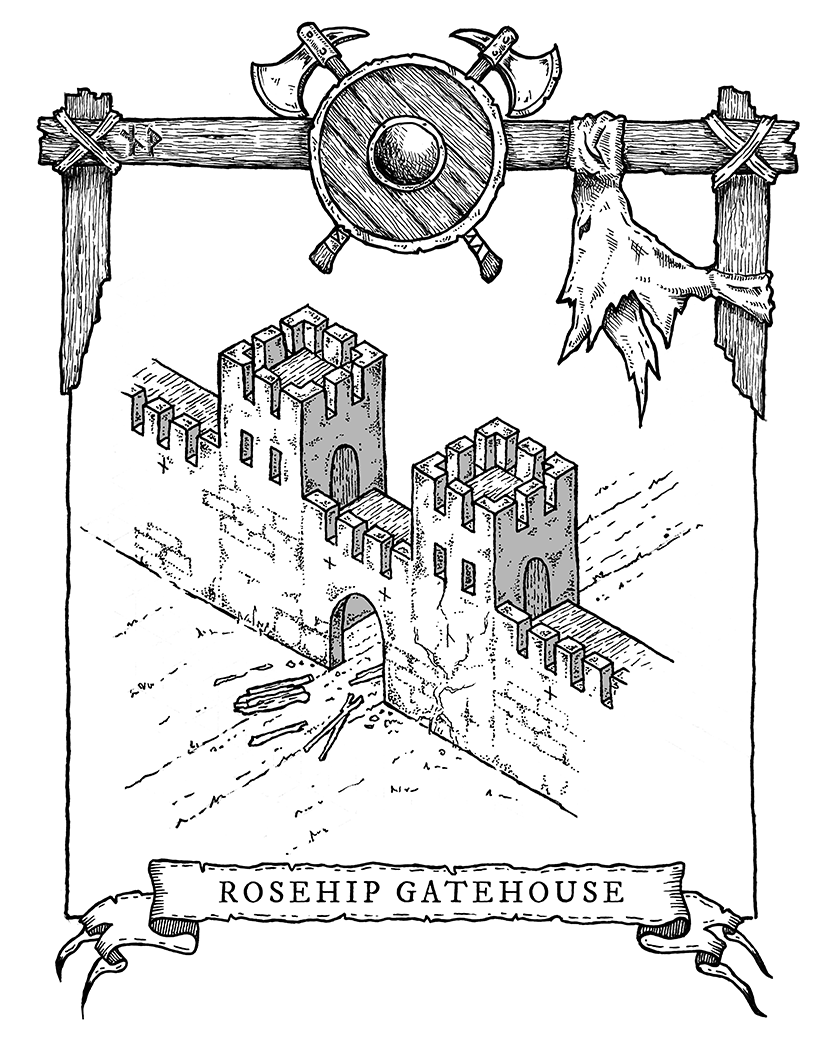A detailed pencil line drawing in black, white, and gray, with a black border, showcases a medieval gatehouse labeled "Rosehip Gatehouse" on a banner at the bottom. The gatehouse features a large, arched entrance without a door, flanked by two square towers rising from either side. The scene includes scattered logs along the path leading through the entrance, suggesting a broken gate. The image is reminiscent of an old advertisement, displaying the fortress-like structure with its evenly peaked towers. The top border imitates rough wood, housing a round shield with two crossed axes behind it and tattered fabric hanging nearby.